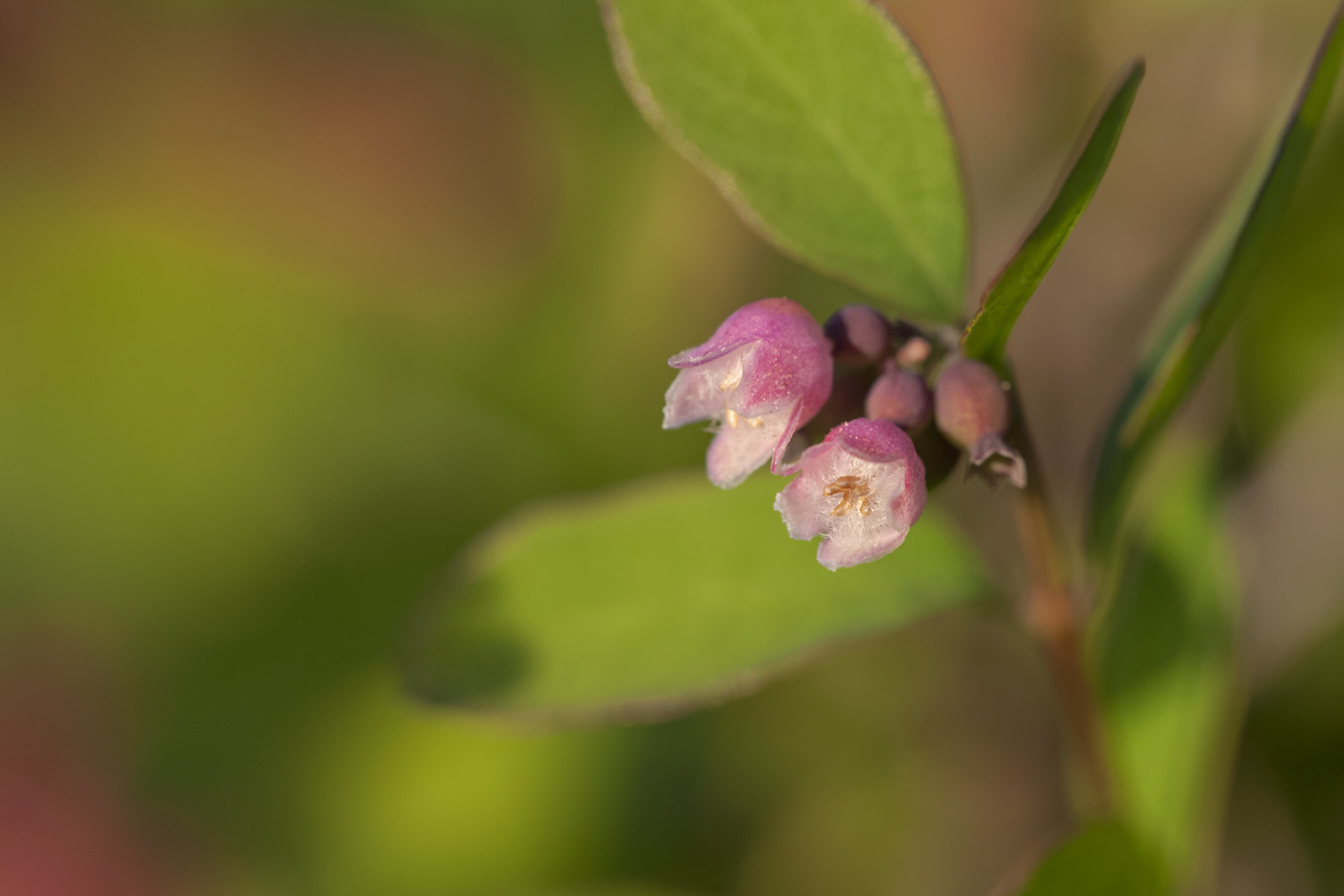This photograph showcases a small cluster of tiny pink flowers on a green stem adorned with green leaves. The image features a very shallow depth of field, rendering the background into a blur of green, which accentuates the sharpness of the flowers in the foreground. The focal flowers are delicate, with a couple not yet open and one in particular pointing slightly down and to the left. These flowers resemble miniature tulips with their pointed, triangular-shaped petals, numbering five or six per bloom. The petals exhibit a gradient from darker pink on the outside to a lighter pink toward the inner part, framing light brown stamens tinged with a touch of gold. Additionally, you can discern more tiny flower buds forming along the brownish-green stem, suggesting new blooms on the horizon. The background blur hints at more greenery and possibly larger flowers beyond the in-focus subjects.